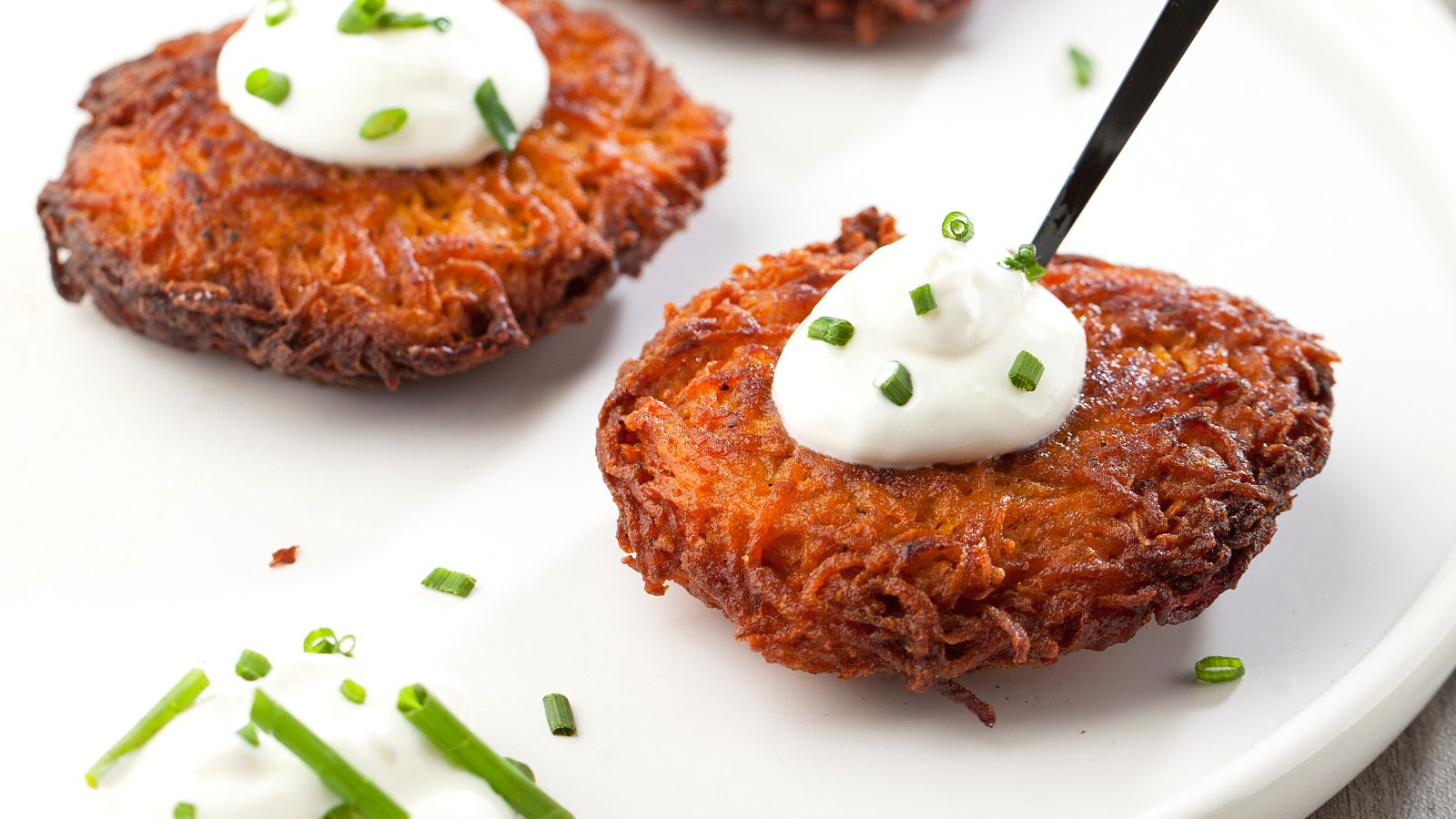This image captures a close-up view of a white plate that almost entirely fills the frame, extending beyond the edges at the bottom and the left side, with just the top right and bottom right corners of the plate visible. On the plate, there are two prominent roundish, brownish-colored patties, which appear to be perfectly fried potato cakes or perhaps potato skins, with a golden, melty layer of browned cheese on top. Each patty has a generous dollop of sour cream in the center, garnished with chopped green chives. A partial view of a third patty is visible towards the top middle of the image, suggesting that there might be more out of frame. Additionally, at the bottom left corner, some extra sour cream with chives extends off the image, possibly for additional dipping. The plate rests on a brownish-grayish tabletop, adding to the rustic presentation of this appetizing dish.